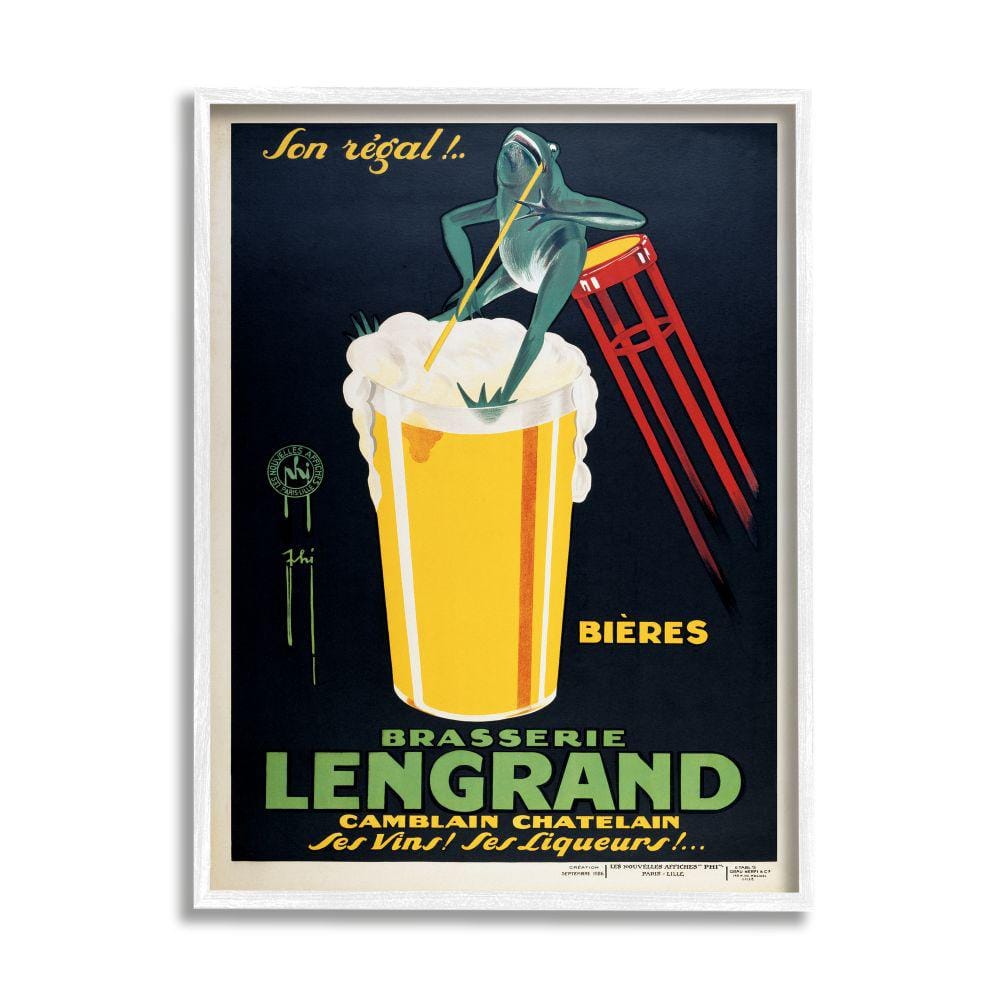This mid-century stylized French advertisement, framed in a simple white border, presents a whimsical scene. The backdrop features a dark blue gradient, seamlessly blending with black accents, and is adorned with vivid green and yellow lettering. Central to the composition is a playful illustration: a large, foamy pint of beer, labeled "B-I-E-R-E-S" in yellow. Perched precariously on the rim of this frothy beverage is a distinguished green frog, seemingly on the verge of toppling over from a small, tilted red and yellow stool. The frog, exuding a sense of regality with a straw in his mouth and his feet propped against the glass, adds a touch of humor to the ad. Overhead, the text reads "Brasserie Langrand," followed by an inviting subtitle, "Camblant Chatelain, c'est vin, c'est liqueur," enticing viewers to enjoy the establishment's wine and liquor offerings. The frog's poised demeanor and the playful arrangement create a charming and inviting portrayal, emphasizing the convivial atmosphere of the restaurant.